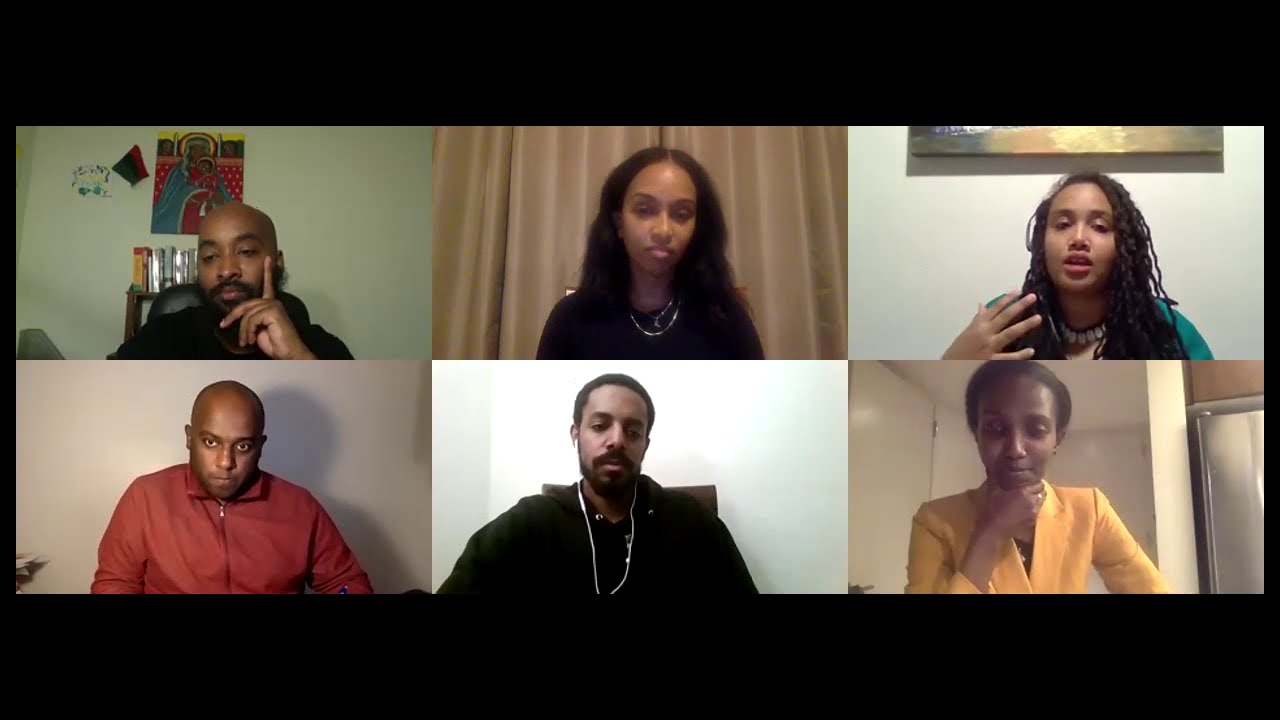The image is a screen capture of a Zoom call featuring six Black individuals arranged in a 2x3 grid. The top row consists of 1) a bald man with a black beard and a black shirt, sitting against a white wall, 2) a woman with long black hair wearing a black shirt and necklace, seated in front of brown drapes, and 3) another woman with braided long black hair and a shell necklace, placed in front of a wall with artwork. The bottom row features 1) a bald man with no beard, wearing a red zip-up shirt against a light background, 2) a man with a black beard, short hair, and wired earbuds, dressed in a black shirt, and 3) a woman with her hair pulled back, wearing a white business suit coat, positioned against a beige background with a visible corner cabinet, resting her chin in her hand. The call is framed by two horizontal black bands, giving the image a pane-like appearance without any text.